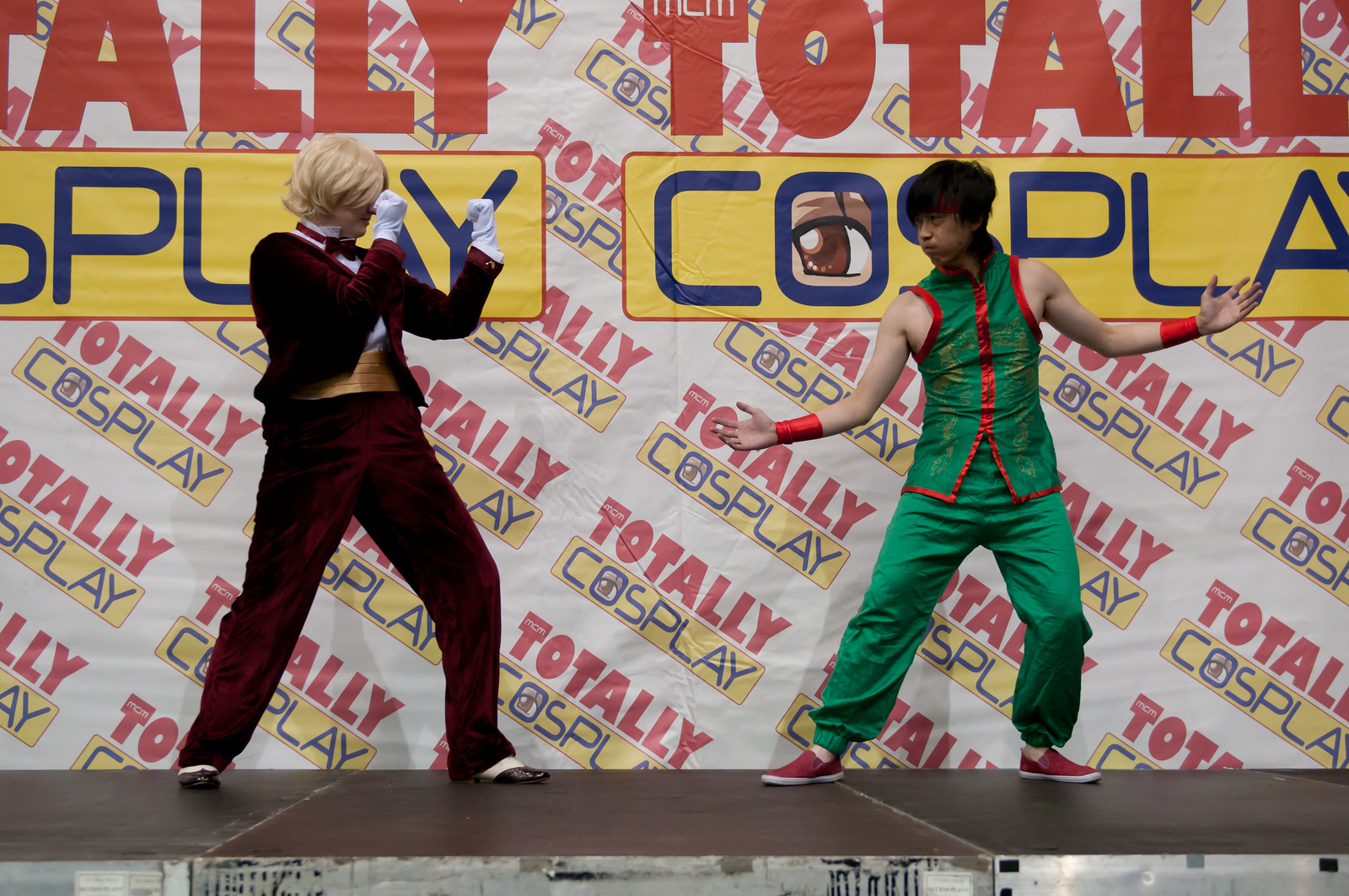The photograph captures a vivid scene on a stage where two individuals are poised in a martial arts stance, facing each other. The backdrop is a wall-sized canvas banner that prominently features the repeated text "Totally Cosplay" in bold red and blue letters on a yellow background. The person on the left, possibly a woman, is dressed in a striking dark red velvet suit paired with white gloves and short blonde hair, which may be a wig. She holds her fists up high, ready to spar. To the right stands a younger gentleman in a green sleeveless vest with red piping, matching green pants, red shoes, and red wrist cuffs. His attire is complemented with black hair. Both individuals appear ready for action against the dynamic and colorful "Totally Cosplay" themed backdrop.